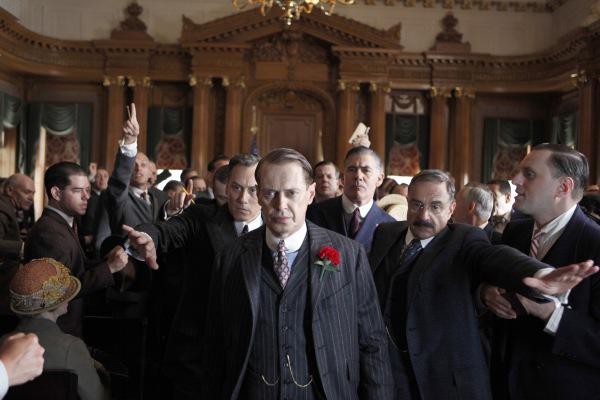The image appears to depict a scene set in the 1940s inside a large, ornately decorated room, possibly a courtroom or a business setting, characterized by tall black shelving, wooden arches, and detailed columns. Centered prominently in the image is a stern-looking man clad in a dark pinstripe three-piece suit, featuring a blue shirt with a white collar, a purple tie, and a red rose pinned to his lapel. Chains on his vest add to his distinguished appearance. This character, moving determinedly through the crowd, is likely played by David Carradine. Surrounding him are numerous men in equally formal business suits, appearing agitated and either raising their hands or attempting to engage with him, while others are holding the crowd back. A woman's figure, notably donned in a stylish hat, is visible seated at the lower left corner, juxtaposed against a man's fist in the same vicinity, contributing to an atmosphere of tension, akin to an old-fashioned courtroom brawl.